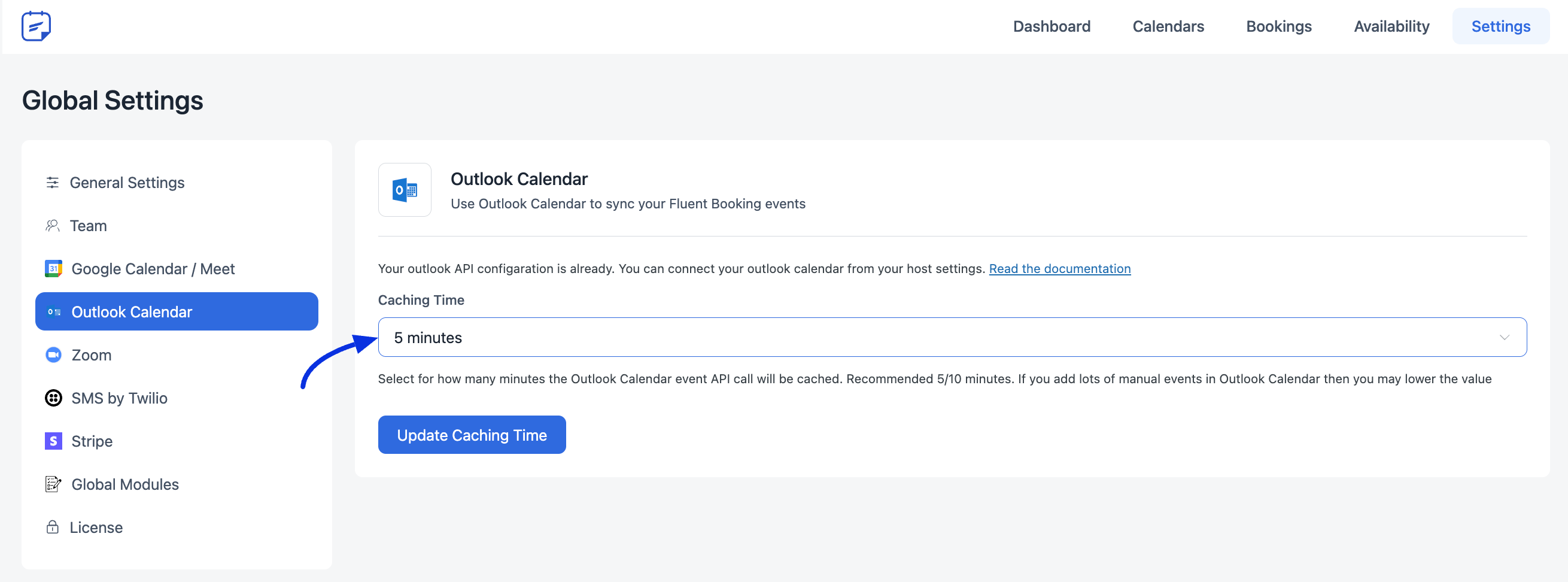The image depicts a detailed interface of a scheduling and calendar synchronization platform. At the top, from the center towards the right-hand side, there is a navigation bar featuring options such as Dashboard, Calendars, Bookings, Availability, and Settings. On the left side, within a gray banner, the text "Global Settings" is prominently displayed. Below this banner, a white box lists various settings options stacked vertically. These options include General Settings and Team, Google Calendar/Meet, Outlook Calendar, Zoom, SMS by Twilio, Stripe, Global Modules, and License.

Currently, the Outlook Calendar option is selected, highlighted in blue, indicating it is active. In the center of the image, the section for Outlook Calendar is expanded, displaying the message: "Use Outlook Calendar to sync your fluent booking events." Below this, it states, "Your Outlook API configuration is already set up. You can check your Outlook Calendar from your host settings or read the documentation," with "read the documentation" being a clickable blue underlined link. 

A caching time setting with a value of five minutes is shown, with a blue arrow pointing upwards towards the text "five minutes." The interface provides guidance, stating: "Select for how many minutes the Outlook Calendar event API call will be cached. Recommended five to 10 minutes. If you add lots of manual events in Outlook Calendar, then you may lower the value." At the bottom, there is a blue button labeled "Update the caching time," offering the user the option to adjust the caching interval.